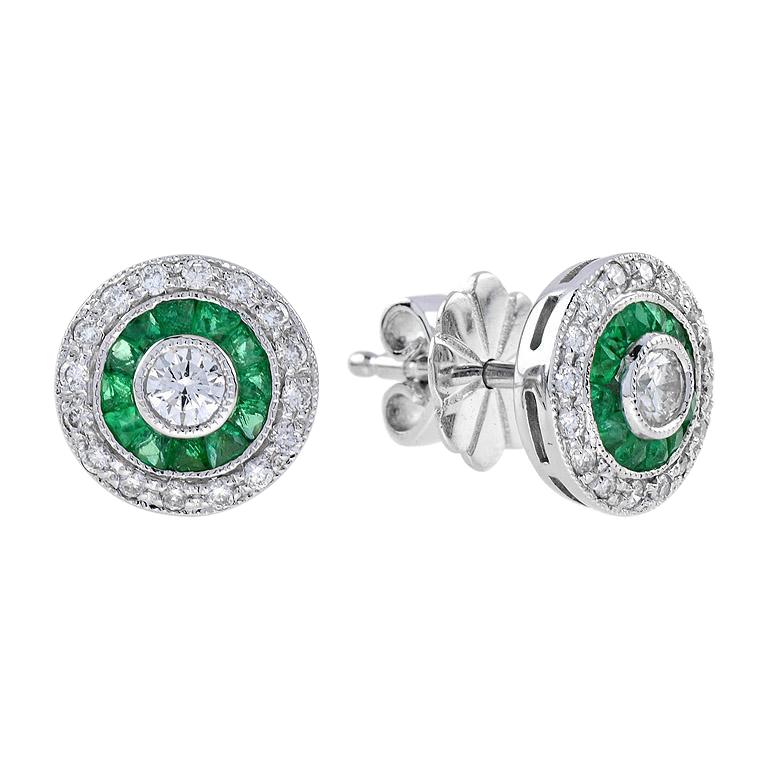The image depicts a pair of matching circular earrings against a white background. The earring on the left is shown from the front, revealing its intricate design: an outer border encrusted with diamonds, a secondary inner border of emerald-green gems, and a large diamond at its center. The outermost part appears silverish. The earring on the right is tilted to reveal the backside, showcasing its silver stem and flower-shaped attachment used for fastening. The attachment is a secure, non-hook style clasp.